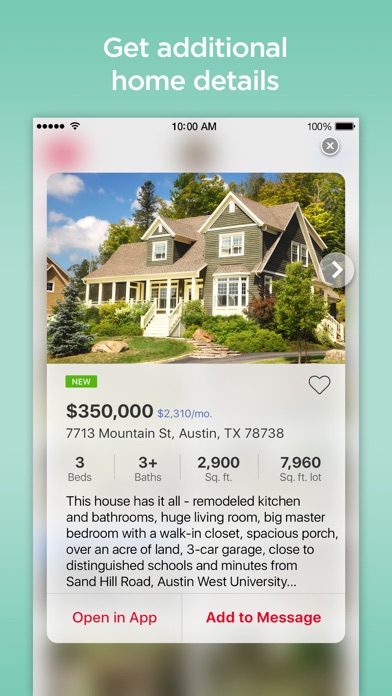### Home Details for Sale: 7713 Mountain Street, Austin, Texas, 78738

Nestled on a lush 7,900 square foot lot, this charming two-story home is now available for $350,000 or approximately $2,310 per month. Located at 7713 Mountain Street in a desirable Austin neighborhood, this property features:

- **House Details**:
  - **Size**: 2,900 square feet
  - **Bedrooms**: 3
  - **Bathrooms**: 3+ (including remodeled kitchen and bathrooms)
  - **Lot Size**: Over an acre
  - **Garage**: Three-car garage
  - **Other Amenities**: Huge living room, spacious porch with white railing, big master bedroom with a walk-in closet, and lots of shrubbery surrounding the house for added privacy.

The exterior of the home boasts gables and a welcoming front porch. A staircase leads up to the main entrance, and from the front porch, there are steps that lead down to street level on a rock staircase. 

The property is located close to distinguished schools and just minutes away from Sand Hill Road and Austin West University, offering convenience and accessibility for families and professionals alike.

For additional details or to schedule a viewing, please open the listing in the app or add it to your message. Don't miss out on this incredible opportunity to own a beautiful and spacious home in the heart of Austin!